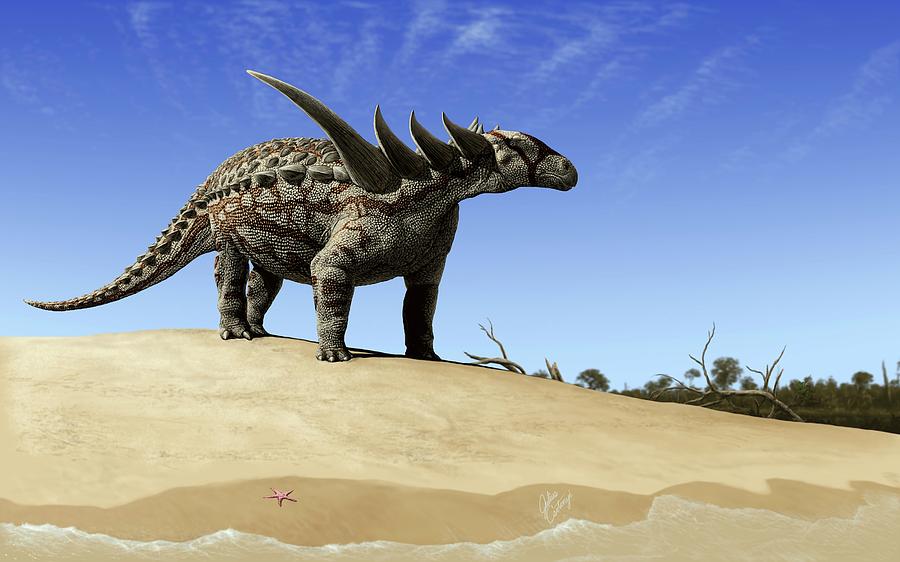This highly detailed, computer-generated illustration in a landscape format depicts a realistic-looking dinosaur standing on a sandy beach. The creature, which resembles a scaled animal with a camel-like pattern of gray and brown, features a narrow snout akin to a horse's head and sports four sturdy legs. It is adorned with multiple spikes: three small ones protruding from its neck and one large spike, in addition to the small spikes covering its body and tail. The dinosaur's skin appears very textured and scaly. In the foreground, the sandy beach is complemented by waves gently washing up and a small pink starfish nestled in the sand. The middle ground reveals sticks and desert-like plants scattered across the beach, with trees in the background. The top portion of the image shows a vast, blue sky dotted with wispy white clouds, adding depth and atmosphere to the scene.